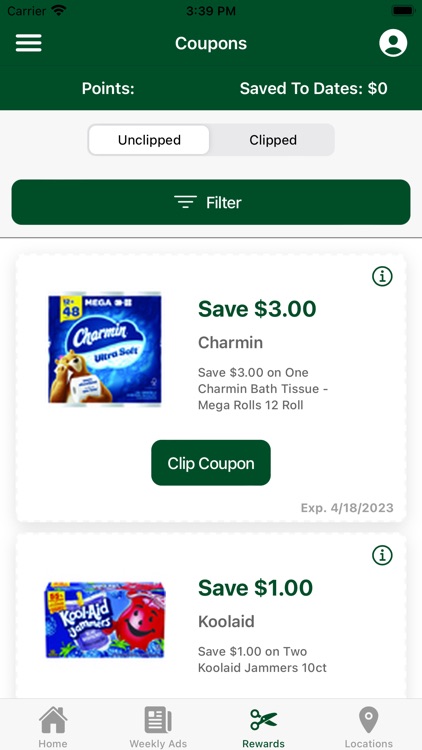The screenshot displays a smartphone interface with various interface elements and coupons. 

### Header Section:
- **Background Color**: Dark green rectangle across the top
- **Carrier**: Displayed in black text
- **Wi-Fi Signal**: All black, indicating strong Wi-Fi connectivity
- **Time**: Centered, displayed as "3:39 PM"
- **Battery Bar**: Appears completely full

### Menu Section (Left Side):
- **Background Color**: White
- **Icons**:
  - Three white horizontal lines
  - "Coupons" text in white next to a white circle, resembling a figure icon

### Points & Savings Section:
- **Text**: "Points ...  Save to Date ...  $0.00"
- **Background**: White

### Filter Section:
- **Button**:
  - **Color**: Dark green
  - **Text**: "Filter" in white, with three horizontal lines that decrease in size downwards
- **Divider Line**: Gray

### Coupons List:
1. **Coupon 1 (Charmin)**:
   - **Image**: Blue package with a bear holding multi-tissue, labeled "48"
   - **Text**: 
     - "Save $3" in green
     - "Charmin" in gray
     - "Save $3 on one Charmin bath tissue mega rolls 12 roll" in gray
   - **Clip Button**: Green box with "Clip Coupon" in white

2. **Coupon 2 (Kool-Aid Jammers)**:
   - **Image**: Blue, likely representing Blue Raspberry flavor
   - **Text**: 
     - "Save $1" in green
     - "Kool-Aid" in gray
     - "Save $1 on two Kool-Aid Jammers ten count" in gray
   - **Clip Button**: Green box with "Clip Coupon" in white

Overall, the interface is organized with a mix of green, white, and gray elements, providing users with various options for filtering and clipping coupons.